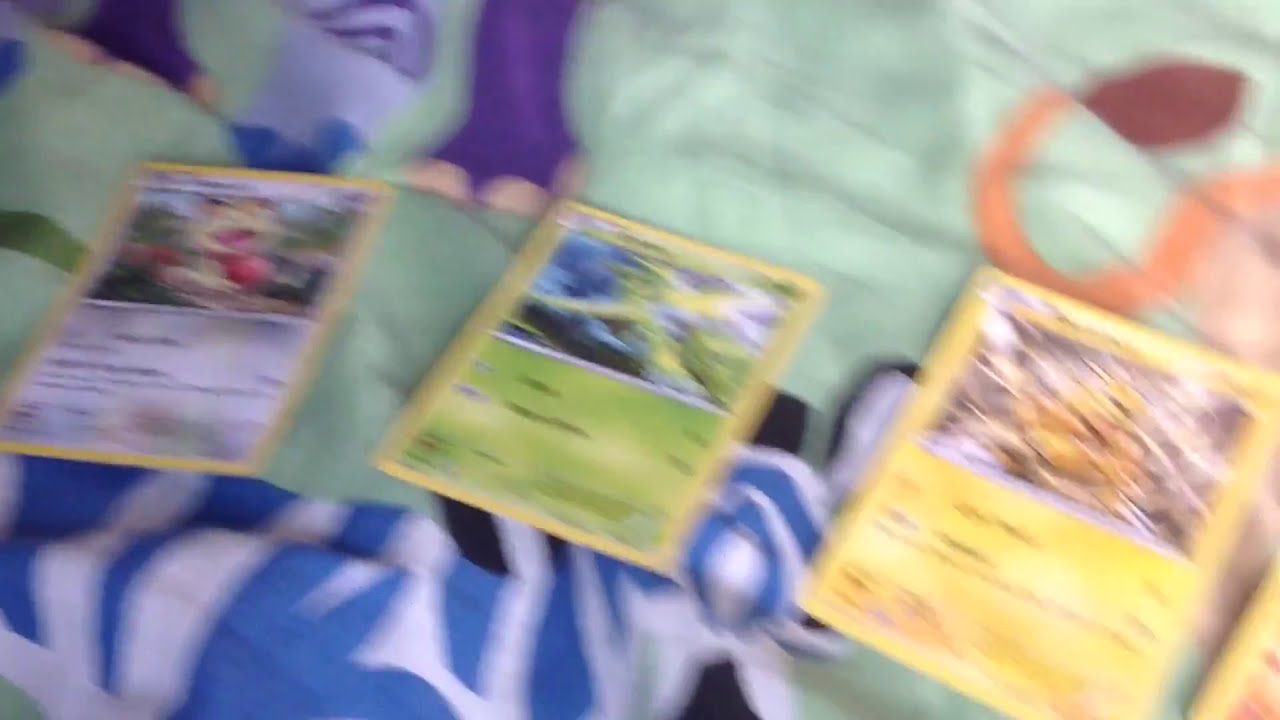The image depicts an extremely blurry photograph, likely taken indoors, showcasing a colorful kid's comforter spread out as the background. The comforter is light green with various blue, white, and orange patterns, including sections of what appear to be cartoon animal designs, such as an orange tail and a purple paw with visible toenails. Centered on this comforter are three distinct Pokemon trading cards, each with a yellow border and varying prominent colors: violet on the left, green in the center, and yellow on the right. Additionally, a partial view of a fourth card is barely visible in the bottom right corner. The Pokémon cards appear to have a similar layout, with a picture on the upper half and textual information on the lower half, although the blur obscures any readable details.